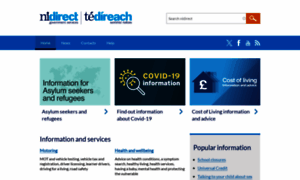The image features an NI Direct logo, with "NI" displayed in blue and "Direct" in light blue. A vertical line separates "NI Direct" from "TED I Reach," where the letter "T" has a diacritical mark above the "E" and appears in blue. "DI Reach" is light blue, also featuring the same diacritical mark.

At the top right, there is a search bar with an orange magnifying glass icon next to it. Below this, there is a navigation menu with a home button that is underlined, indicating it is the current selection. Three additional menu options are present but appear blurred and unreadable.

Further down are icons linking to various social media platforms, including Twitter, Facebook, and two others. This section is located just below the search bar area.

The main content area highlights three articles, each accompanied by an image and a brief description:
1. The first article on the left is titled "Information for Asylum Seekers and Refugees," featuring an image of a globe. It provides information services for asylum seekers and refugees.
2. The middle article is "COVID-19 Information," showcasing an illustration of the COVID virus with a magnifying glass. It offers details on how to find information about COVID-19.
3. The last article is titled "Cost of Living," displaying a house with a euro symbol. It offers information and advice on living expenses.

The overall background of the image is white, creating a clean and simple backdrop for the content.